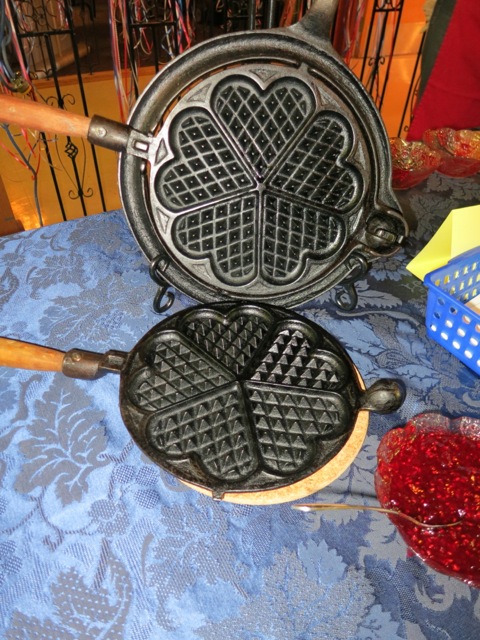This close-up, color photograph, taken in portrait orientation, features an old-fashioned, cast iron waffle maker as its central focus. The waffle maker, with its distinct clover-like pattern composed of five heart-shaped sections, is open to reveal its clean, intricately designed interior. It sits atop a medium blue tablecloth adorned with a floral, lacy pattern, adding a touch of elegance to the setting. The waffle iron has dark brown handles with metal tips, indicating its functionality and sturdy design. To the right, there’s a bowl containing a red, jelly-like substance, presumably raspberry jam or compote. Additionally, a blue plastic basket containing some paper is visible in the background, while wrought iron gatework can be faintly observed in the distance, further adding to the scene's rustic charm.